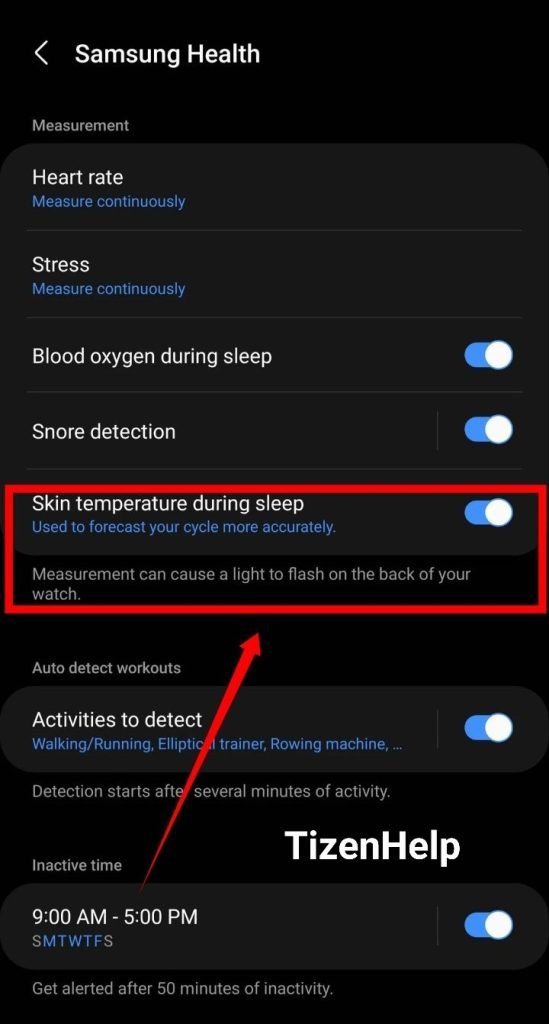Screenshot of Samsung Health app, showcasing various tracking features on a mobile device:

1. **Measurement Settings**:
    - **Heart Rate**: Displayed at the top position, with an option to measure continuously highlighted in blue text.
    - **Stress**: Located in the second row, also featuring a continuous measurement option in blue text.
    - **Blood Oxygen During Sleep**: Toggled on, indicated as active.
    - **Snore Detection**: Also toggled on, showing it is functional.
    - **Skin Temperature During Sleep**: Toggled on and highlighted with a red box and a red arrow pointing upward, emphasizing its importance.
    
2. **Auto-Detect Workouts**:
    - **Activities to Detect**: Lists walking, running, elliptical training, and rowing machine, all toggled on for automatic detection.

3. **Inactive Time**:
    - **Schedule**: Set from 9 a.m. to 5 p.m. on Monday, Wednesday, Thursday, Friday, and Saturday, with the feature toggled on.
    - **Alert**: Notification settings to alert the user after 15 minutes of inactivity.
    - **Tizen Help**: Positioned above the inactive time, providing assistance or information related to Tizen.

The red arrow originating from the "Inactive Time" section aims at the "Skin Temperature During Sleep" measurement, accentuating its critical role in the user’s health monitoring setup.